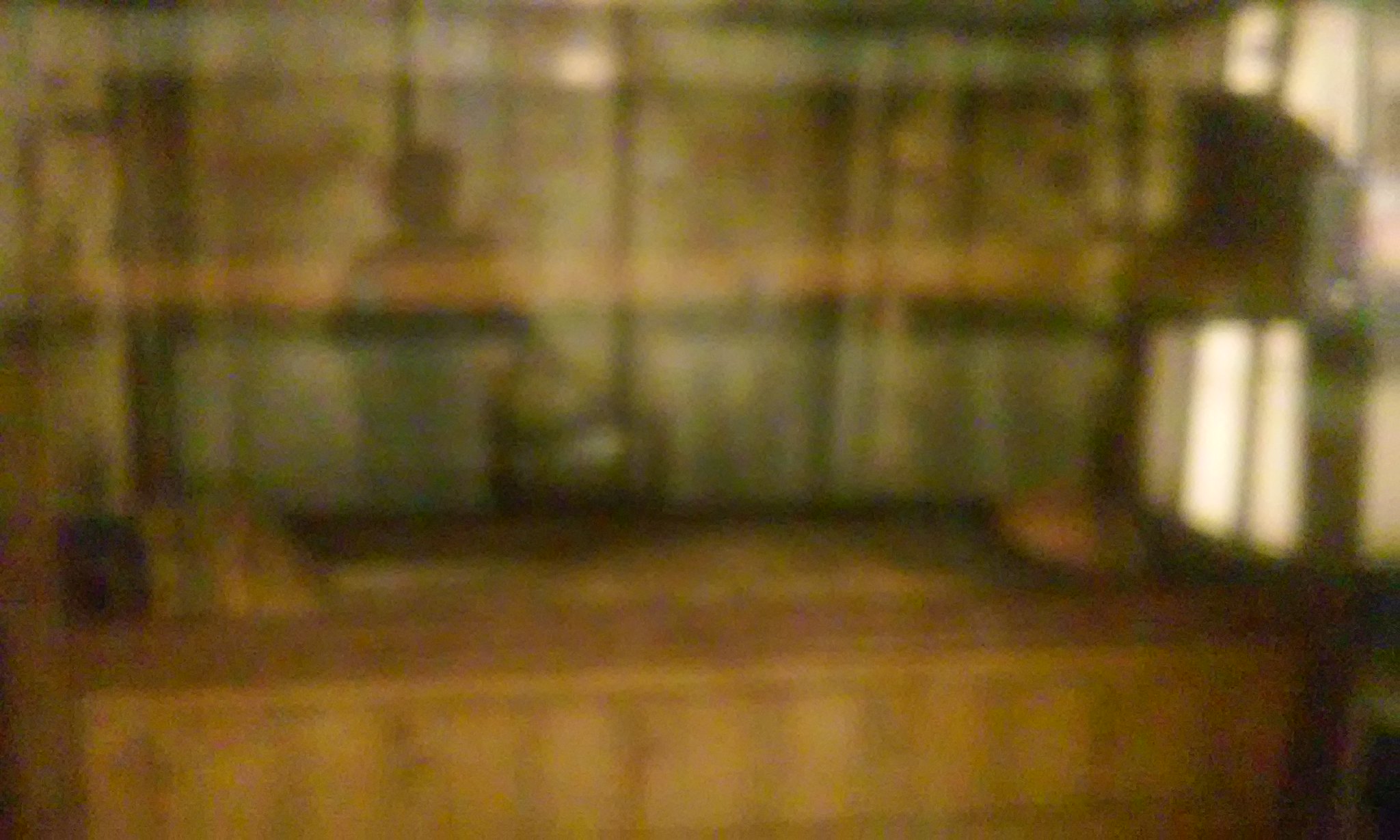The image is fairly blurred and of very low quality, making it difficult to discern exact details. However, it appears to depict the interior of a room with a large, dark brown table or desk in the foreground. The table exhibits varying shades of dark, drab brown and has a few indistinguishable items on it, possibly a bottle and a couple of books. The background of the image includes a slightly greenish wall, where the shadow or silhouette of a person is prominently reflected. This shadow is near the left center of the image, indicating the presence of a glass window or mirror on or near the table. To the right, multiple rectangular beams of light are visible, suggesting another light source or a window. The overall scene is very out-of-focus, making it difficult to determine if the setting is inside a building, such as a storefront or shop, or another type of interior space.